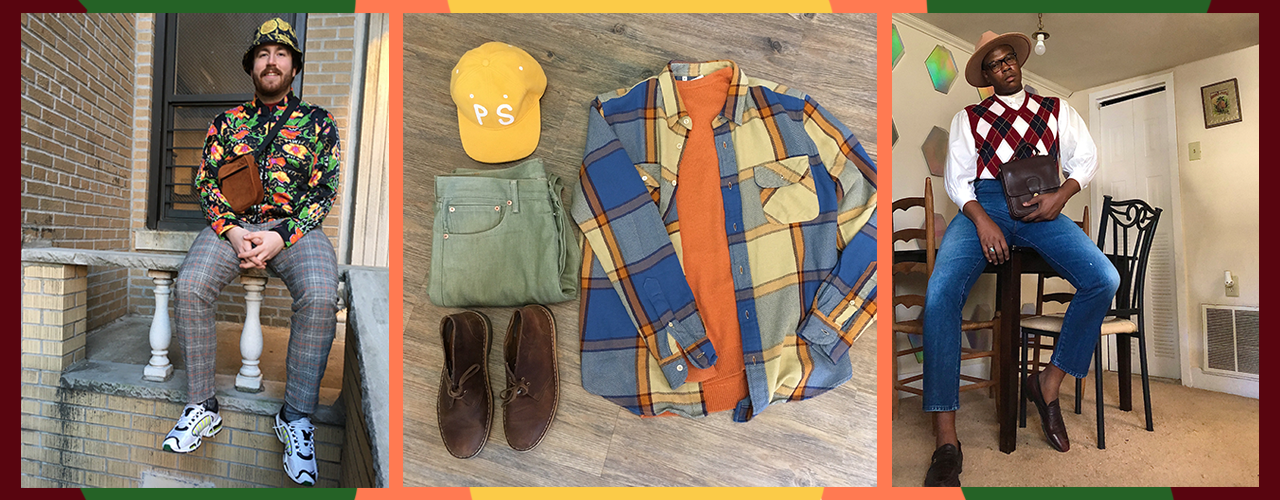The image consists of three distinct photographs arranged in a collage, framed by a maroon border with green and yellow accents. The photo on the far left features a man sitting on a porch railing outside a brick house. He dons a vibrant, multi-colored long-sleeved shirt with black, green, red, and yellow patterns, paired with grayish plaid pants and sneakers. A hat matching his shirt's yellow pattern sits atop his head, and a brown satchel rests on his shoulder. In the center is an assortment of clothing displayed on a wooden floor, including a blue and beige plaid shirt layered over an orange t-shirt, green pants, brown suede shoes, and a yellow baseball cap with "P.S." embroidered on it. The rightmost photo shows a man in a sweater vest, blue jeans, and dress shoes, sitting on the edge of a kitchen table in a room with beige walls. He sports a round-brimmed hat, glasses, and holds a leather satchel. The overall composition of the images, including the frames with their varying colors, suggests a fashion catalog layout showcasing a diverse array of stylish outfits.